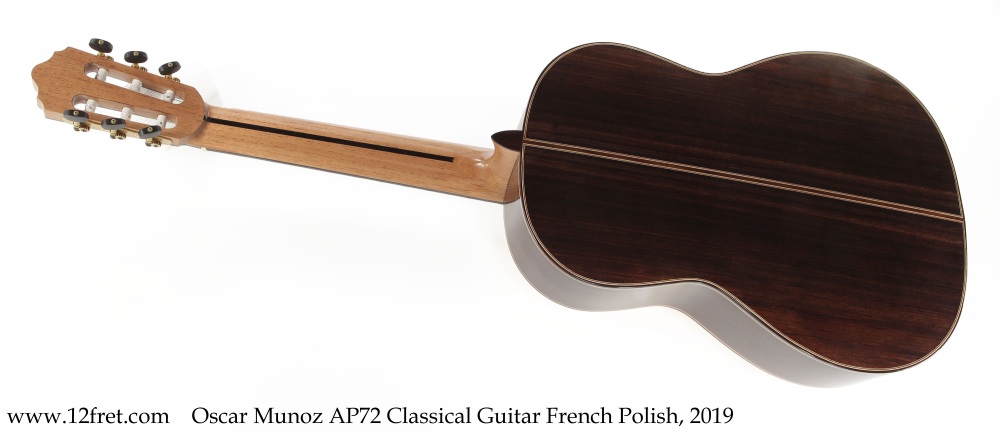This image showcases the back of an Oscar Munoz AP-72 Classical Guitar, finished in French Polish from 2019. The main focal point is the body of the guitar, crafted in a rich dark brown wood with a maple neck and headstock in a lighter tan hue. The background is entirely white, emphasizing the guitar without any distracting elements or surfaces. At the bottom, the text reads "www.twelvefret.com," followed by "Oscar Munoz AP-72 Classical Guitar French Polish 2019." The guitar features notable details such as downward-facing tuners and a visible truss rod notch on the back of the neck. Though the front and strings are not visible, the craftsmanship and classical aesthetic are clearly showcased.